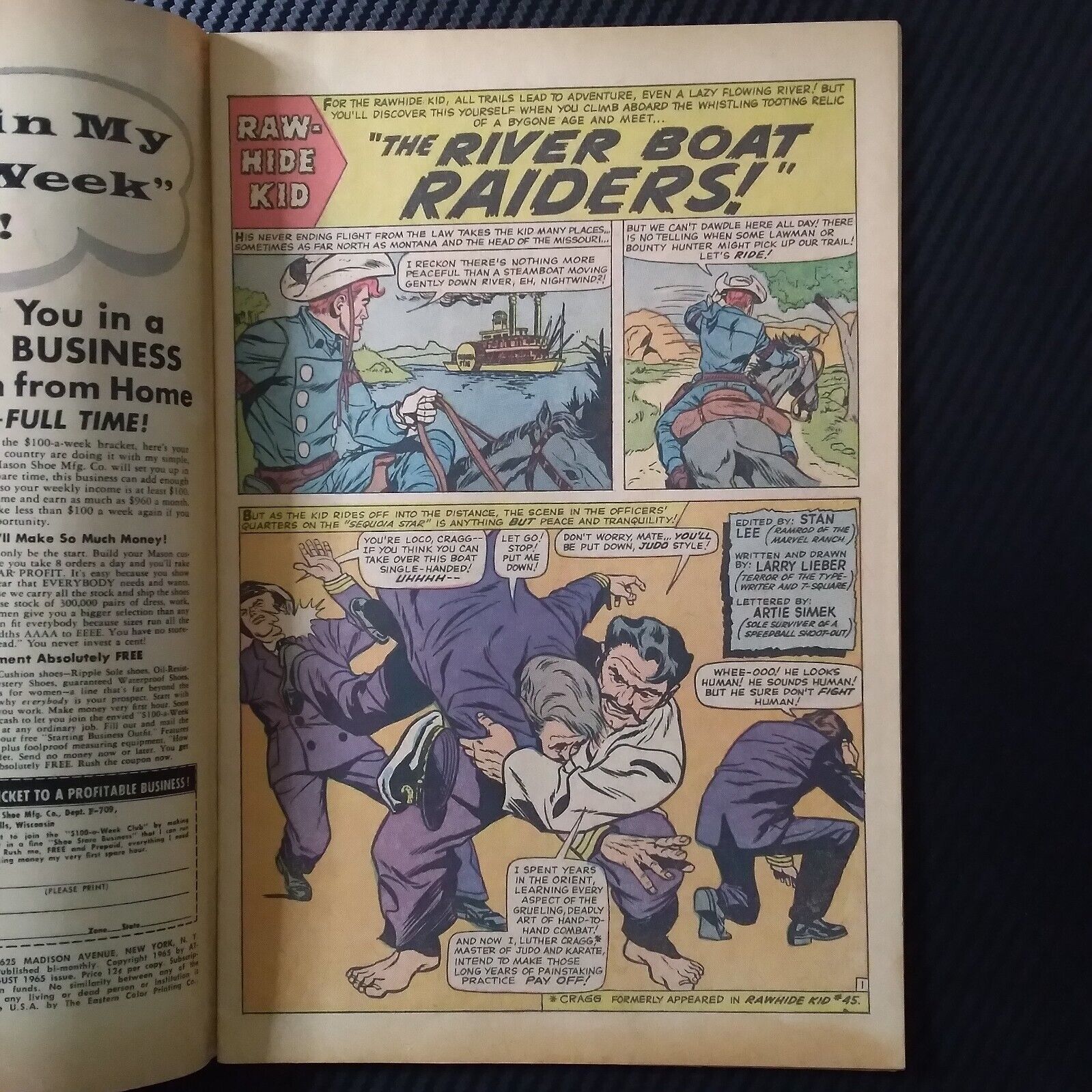The image shows a comic book page titled "The Riverboat Raiders," featuring vibrant yellow, red, blue, purple, and orange backgrounds typical of comic books with various sized panels. It lies open on a plain black surface. At the top, a yellow rectangle with a red arrow holds white text reading "Rawhide Kid." Below it, the title "The Riverboat Raiders" is displayed within the yellow rectangle, with an introductory text hinting at the Rawhide Kid's adventures leading to a steamboat on a lazy flowing river. 

The first panel shows a man in a blue suit on a horse, looking towards a steamboat on a river. In another panel, the same man rides away on his black horse. The bottom half of the page is dominated by an intense fight scene: a large, bearded man in a white shirt executes a judo throw on another man in a purple suit, while two additional men in purple suits are also involved in the brawl. In the background of the fight scene, the Rawhide Kid rides off into the distance. Part of an advertisement for a home business opportunity is visible on the adjacent page.